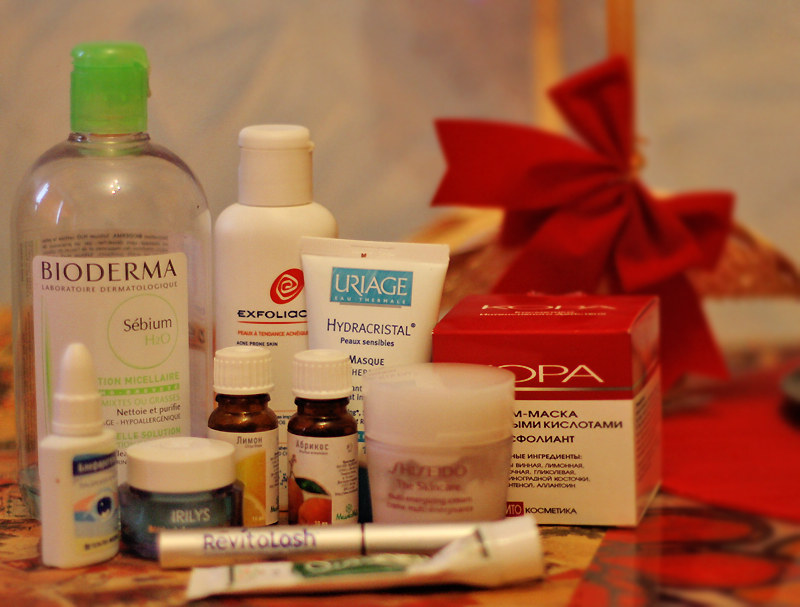A vibrant photograph showcasing a diverse array of skincare and cosmetic products artfully arranged. The scene features several bottles and packages of varying shapes and sizes, each adorned with writing in different languages. Among the collection, there is a clear bottle with a green cap, a sleek white bottle, and a striking red one. Adding to the aesthetic appeal, a delicate ribbon graces the background, while the products rest elegantly on a bold red countertop. In the foreground, a tube labeled 'Revitalash,' likely a mascara, captures the viewer's attention. The image beautifully blends elements of beauty and care, presented in a visually captivating manner.